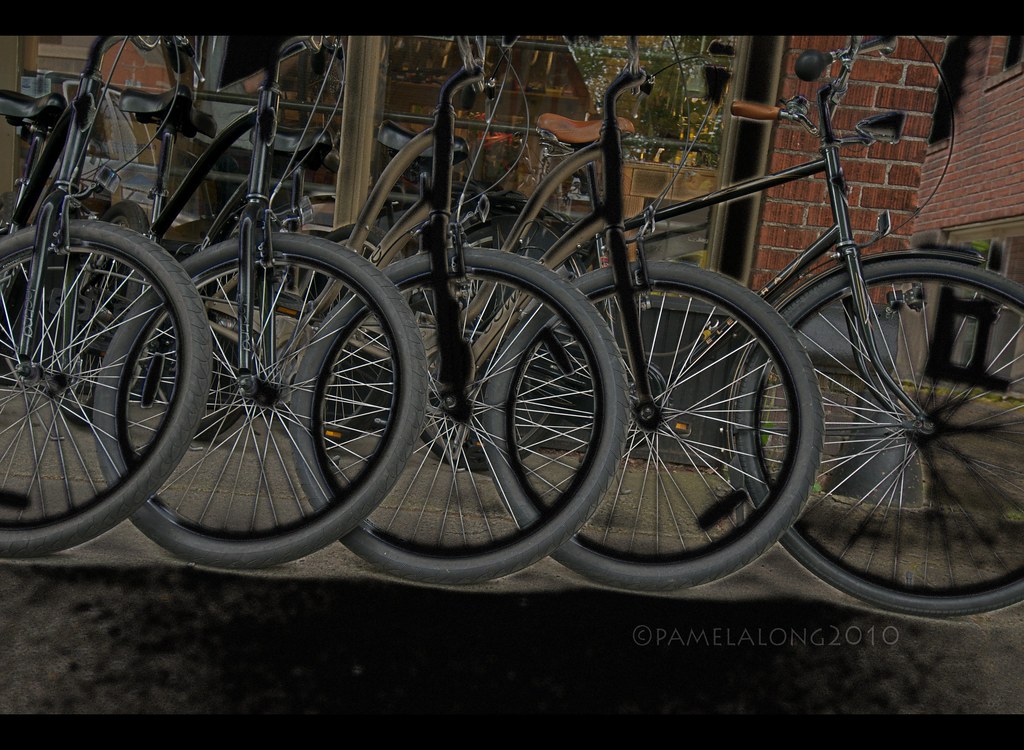This horizontal digital collage or digitally enhanced photograph, created by Pamela Long in 2010, features five black hybrid bicycles perfectly aligned side-by-side, their fat, whitish tires and bright chrome spokes facing the camera. Central to the image, the bicycles' dark bodies extend up to their handlebars, with the first bike on the right notably equipped with a black and silver squeeze horn. One of these bikes sports a distinctive brown leather saddle, contrasting the black leather saddles on the others.

The artistic enhancement makes the wheels appear almost artificial, with shimmering gray tires and prominent white spokes creating a striking visual effect. The bicycles’ nearly monochrome appearance, with dark tones dominating, gives the image an almost negative-imposed look. The background showcases a red brick building with large floor-to-ceiling windows, a smaller window with black bars, and a green column. Additional details in the background include visible red roofs and splashes of greenery, lending a hint of the surrounding environment. The photo carries a watermark along the bottom, marking it with the artist's name and the year of creation.